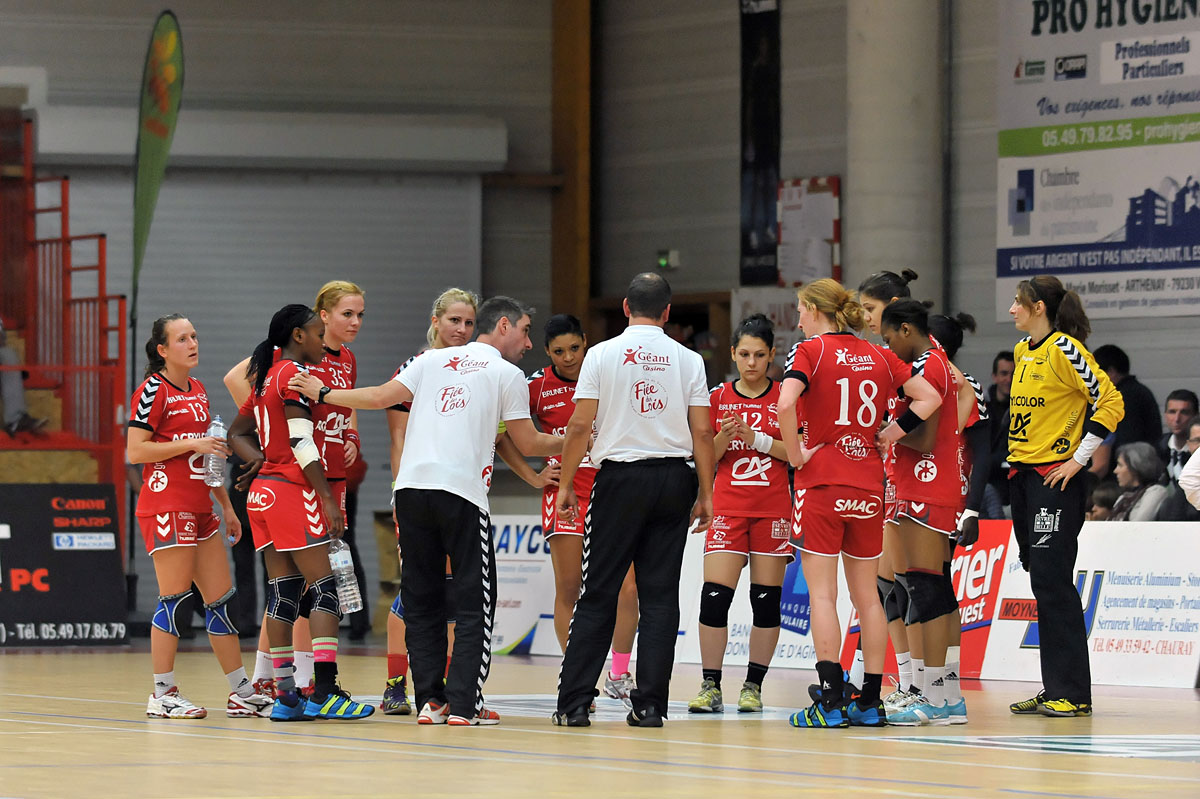The image depicts a high school girls' volleyball team during a sporting event in a gym. The team is dressed in red uniforms consisting of red tops and shorts, complemented by a variety of colored athletic shoes and knee pads in black and blue. They are gathered in a huddle on a hardwood basketball court, likely receiving instruction from two men, presumably coaches, who are dressed in white t-shirts and black pants. An older woman, possibly a staff member or another coach, stands to the right in a yellow top and black pants, observing the scene. The gym is detailed with distinguishable features such as a large white garage door in the background, red bleachers on the left filled with spectators, and various advertisement banners and signs along the sides, including one that reads "Gient Casino" and another partially visible sign that appears to say "Fire De Lois." The gym floor exhibits white and blue lines indicative of volleyball court markings.